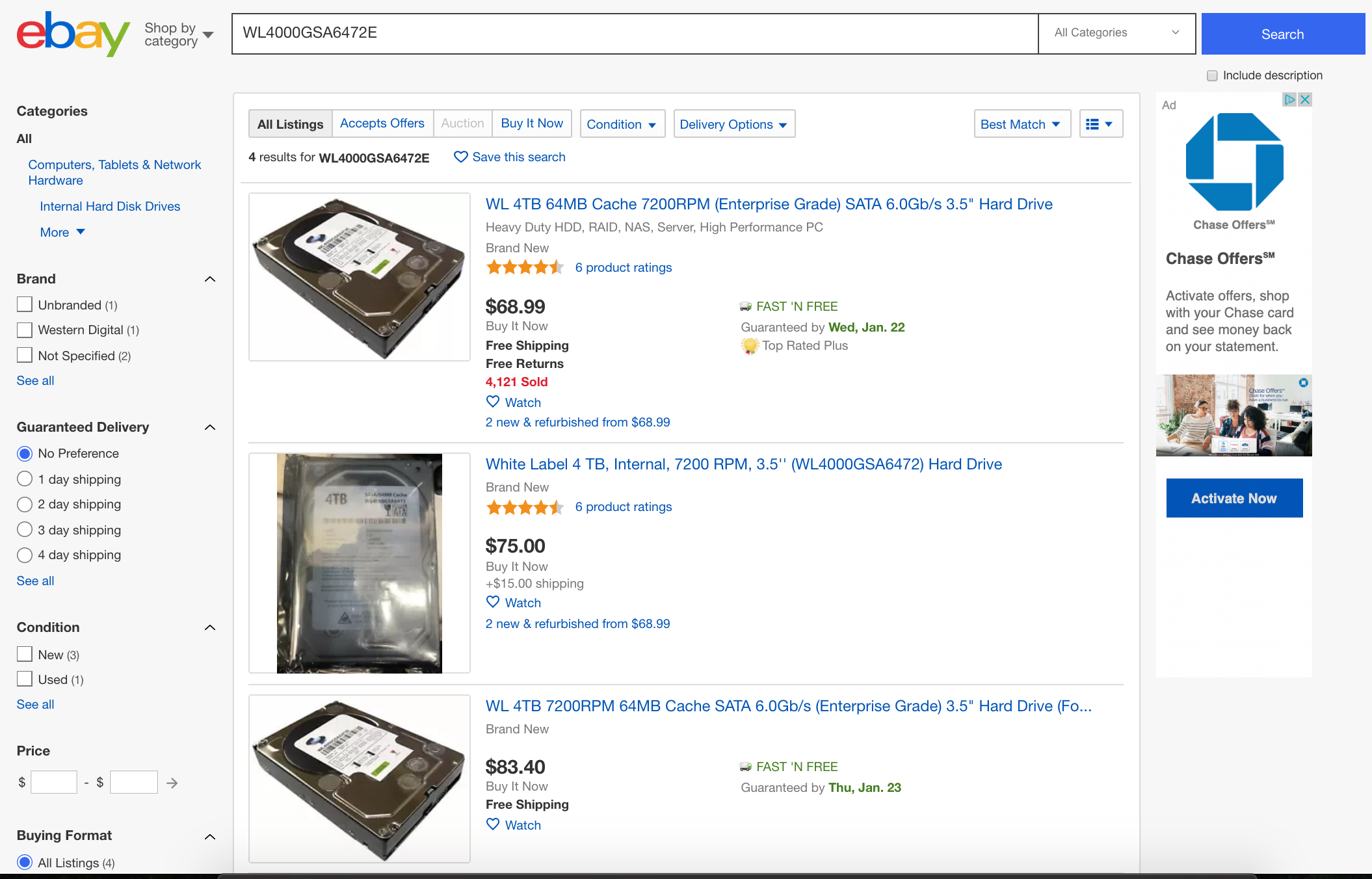### Detailed Caption:

The image depicts a webpage with a blue background, primarily showcasing the eBay website. At the top of the page, the eBay logo is displayed prominently with a red "e", blue "b", yellow "a", and green "y".

Directly below the logo, there's a section labeled "Shop by Category," which includes a large search box. Next to the search box is a drop-down menu labeled "All Categories" with a down arrow, followed by a blue "Search" button.

On the left sidebar, there are various filtering options:

1. **Categories**: Includes options such as "Computers" among others, with a down arrow indicating more categories.
2. **Brand**: Lists three different brands with checkboxes beside them and an "up" arrow, followed by a "See All" link in blue.
3. **Guaranteed Delivery**: Offers five choices, each with a checkbox beside it. The option "No preference" is highlighted in blue, accompanied by an "up" arrow.
4. **Condition**: Provides options for "New" or "Used" with corresponding checkboxes and an "up" arrow at the end, followed by the "See All" option.
5. **Price**: Includes input boxes for "Starting Price" and "To Price."
6. **Buying Format**: Features a blue button labeled "All Listings."

A long black line divides the above content from the main section below.

In the main content area, there's a large white box at the top with filter tabs including "All Listings," "Auctions," "Offers," "Buy It Now," "Condition," "Delivery Options," and "Best Match." Below these tabs is a sorting box with a small blue line, three little blue lines, and a down arrow.

The first listing is for a "WL-4TB-64MB Cache 7200 RPM Enterprise Grade SATA 6.0 GB 3.5" Hard Disk," priced at $66.99 with free shipping and returns. The product has sold 4,121 units and features a heart icon indicating it can be added to a wish list. The product description continues with "White Label 4TB Internal 7200 RPM 3.5 Inch Hard Drive," rated at 4.5 stars.

The second listing is for a "WL-4TB 7200 RPM 6.4 MB Cache SATA 6.0 GB Enterprise Grade 3.5 Inch Hard Drive," priced at $83.40 with free shipping. This listing also features a heart icon labeled "Watch" and a box marked "Fast and Free," indicating delivery by Thursday, January 23rd.

On the right, a small section at the top includes a word with a tiny box next to it, followed by a long white box with the option to "Add." Below two blue X-marked boxes, there's a blue shape labeled "Choose Office" or "Chase Offers," which states "Activate Now." At the bottom of this section, there's a blue button.